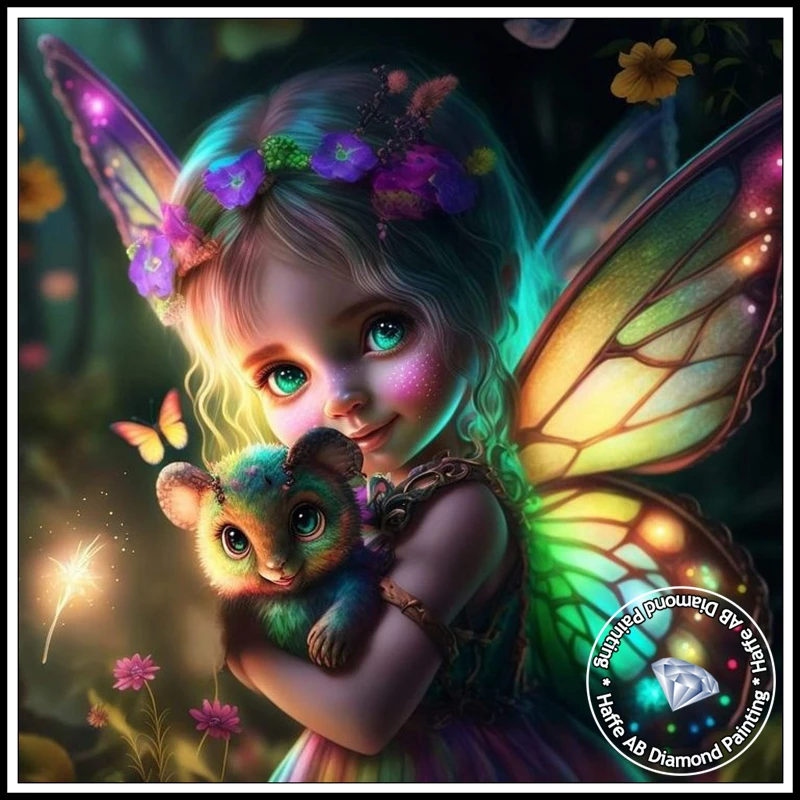This intricate digital artwork features a young fairy reminiscent of Tinkerbell from Peter Pan, complete with a charming set of wings on her back and an additional wing seemingly floating behind her head. Showcasing bright green eyes and adorned with blonde hair intricately detailed, she is dressed with flowers perched on top of her head. The image exudes a whimsical, neon-colored ambiance akin to a children's book illustration. She cradles a small, fantasy creature that appears to have multiple fingers, indicating an AI-generated origin, with her own fingers curiously missing. A butterfly or perhaps a dragonfly flutters next to her, and other flowers, both golden and pink, float in the background, adding layers of enchanted detail. The illustration is branded with "A-F-F-E-A-B Diamond Painting," encircled twice with a white outline, positioned at the bottom right corner. The backdrop features soft, out-of-focus elements, enriching the artwork's enchanting atmosphere.